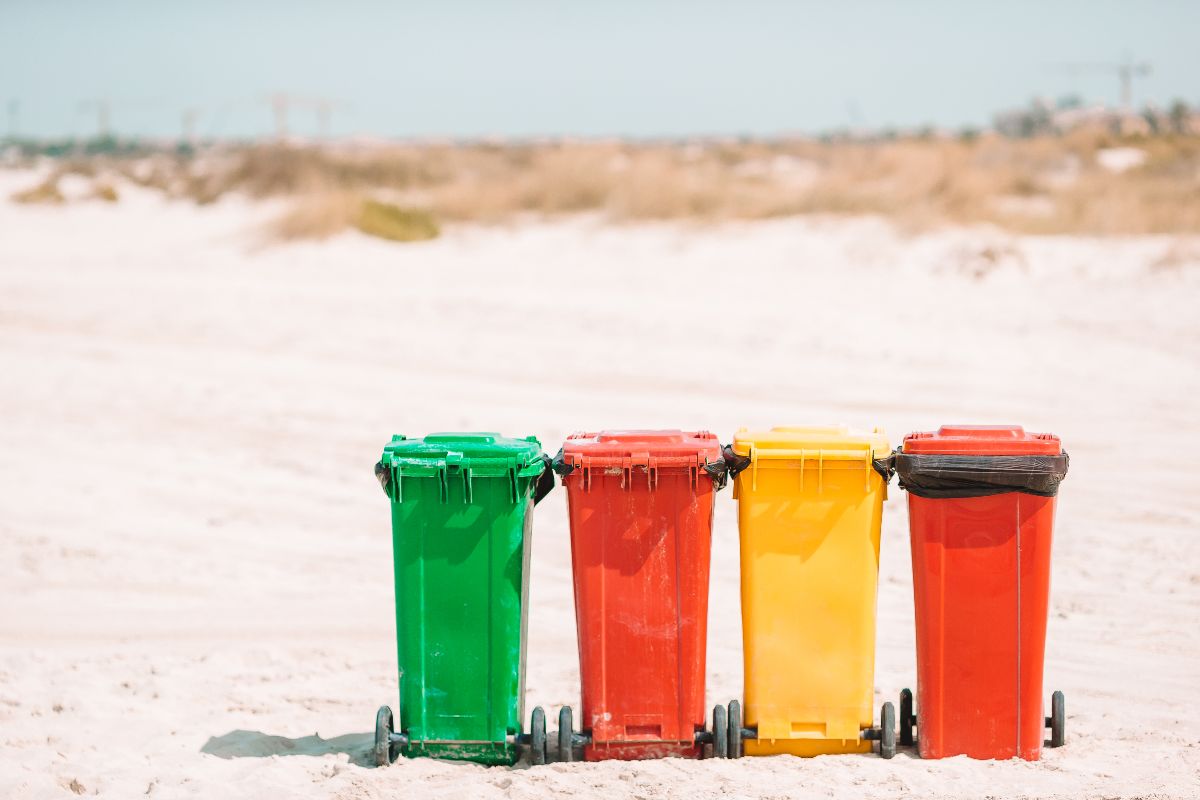A horizontally aligned rectangular picture captures four waste bins standing in a row on a light tan, sandy beach. The bins, which are plastic and equipped with black wheels and lids with black trash bags peeking out, are aligned at the bottom center of the image. From left to right, the bins are colored green, orange, yellow, and orange. We're looking at the backsides of the first three bins, while the fourth shows its front with a visible brown handle. The sand extends to a band of brown grass, and beyond that a blurry, overcast sky. In the far distance, barely discernible through the blur, are possibly some green trees and electrical wind turbines. The beach is devoid of people, and the overall image lacks text or a border.